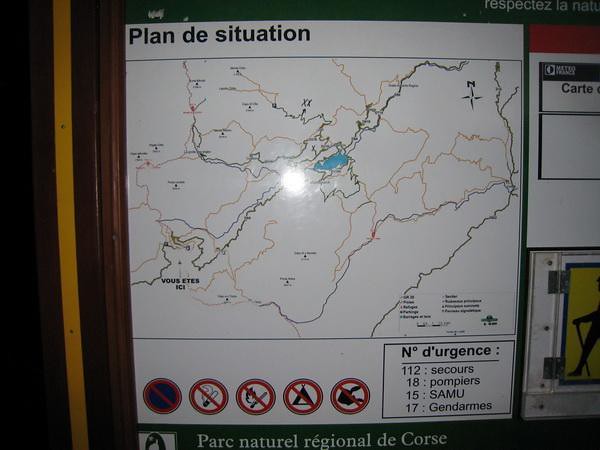The photograph depicts a detailed map mounted on a whiteboard, with light reflecting off its center. The map is primarily in French and titled "Plan de Situation" at the top. At its center, there is a small blue lake surrounded by various trails. Several areas on the map are marked, and beneath the map, numerous cautionary symbols such as red circles with crosses through them indicate prohibitions: no smoking, no campfires, no camping, and possibly no hunting. Additional text below these symbols reads "Parc Natural Regional des Corses," and above this description are emergency contact numbers in a black box, including: "North D'Urgency 112, Secours 18, Pompiers 15, Samu 17, Gendarmes." The map is set against a brown wall with a yellow vertical strip visible on the left, and to the right edge of the photo, there are two other partially visible posters. The room appears darkened, emphasizing the map's details and the reflective light.